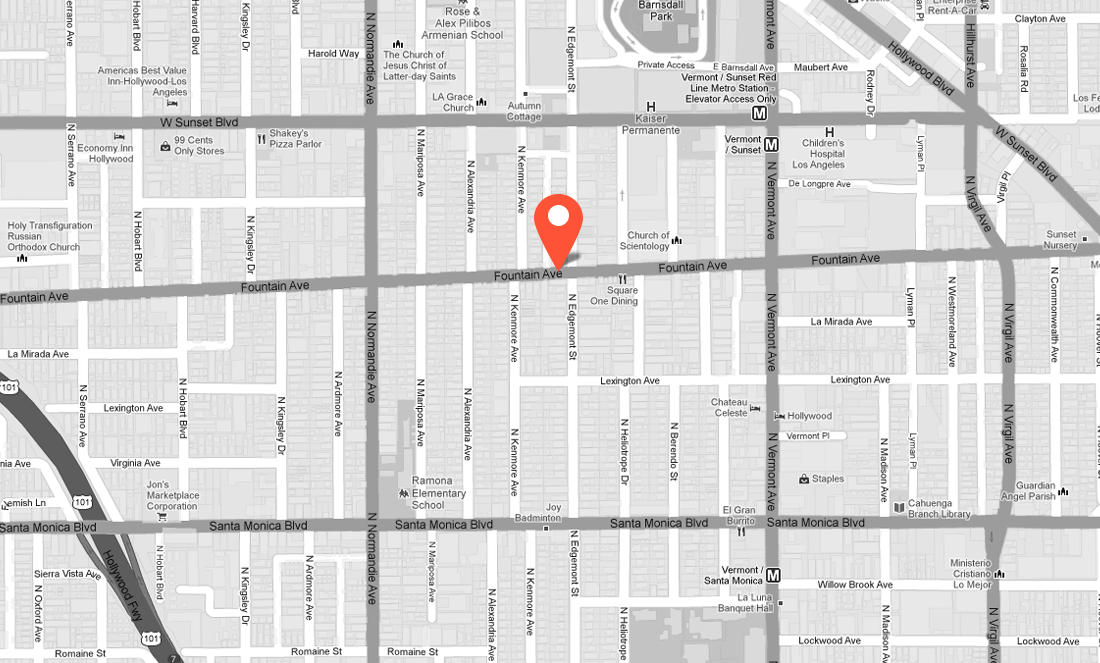A detailed Google Maps image depicts an urban grid featuring three prominent east-west streets: West Sunset Boulevard at the top, Fountain Avenue in the middle, and Santa Monica Boulevard at the bottom. Intersecting these thoroughfares are three notable north-south streets, forming a structured network. On the map's southwest corner, a diagonally-oriented, larger road marked as Highway 101 cuts through the area, while the northeast corner features another diagonal street labeled Hollywood Boulevard, running from southeast to northwest. These major streets are highlighted in dark gray, contrasting with a multitude of smaller, connecting streets shown in white, creating a dense pattern typical of urban centers. The entire image is monochromatic, except for a prominent red marker, shaped like a teardrop with a solid white circle at its peak, indicating a specific location. This pin points precisely at the intersection of Fountain Avenue and a smaller, unnamed street, suggesting a focal point within the intricate street grid.